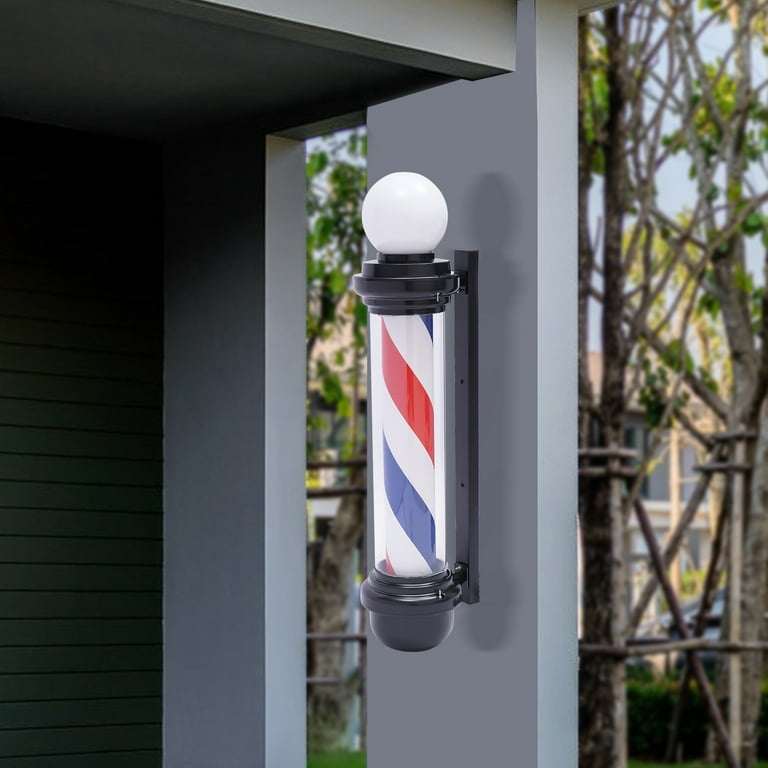The image showcases a digitally rendered barbershop sign that is prominently mounted on a gray wall in a portrait-oriented frame. The sign features a classic barber pole with its iconic red, white, and blue swirling stripes encased in a cylindrical tube, suggesting the potential for motion. The pole is capped with a white ball at the top, with both ends bracketed in black. This gray wall is part of an exterior setting with two identical sections and a window between them. To the left, there's a dark green paneled wall. In the background, a cluster of thin trees with brown trunks and sporadic green and yellow foliage rise against a very light blue sky, which hints at other indistinct buildings further away. The overall scene is tranquil, reflective of a typical streetscape wherein this familiar barbershop element serves as a focal point.